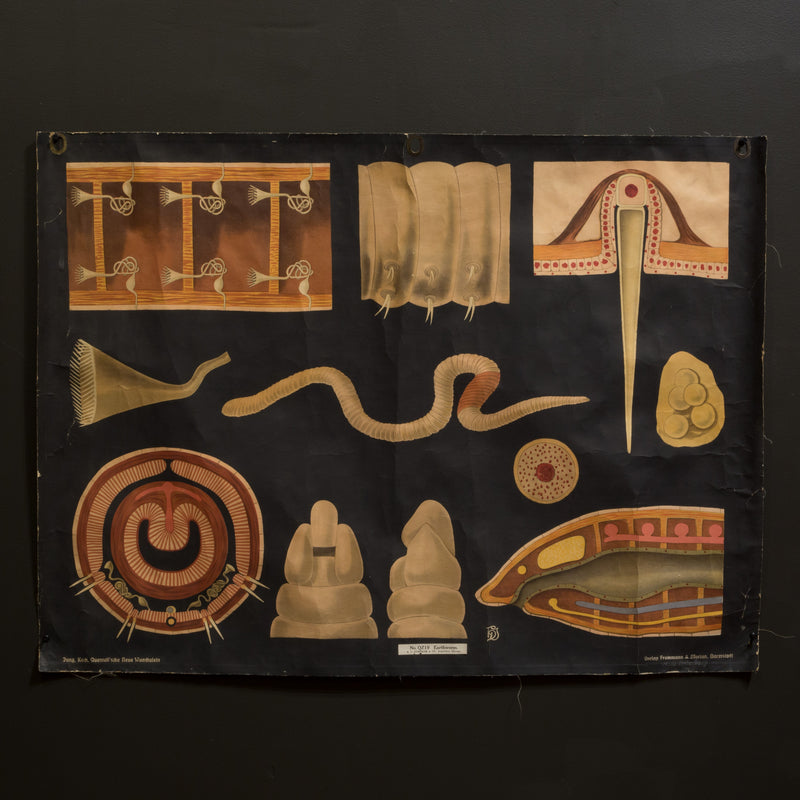The image is a detailed scientific illustration depicting an earthworm, comprising about eight to ten individual sections arranged on a black background. Each section is intricately designed, showcasing various aspects and cross-sections of the earthworm's anatomy. Most of the images feature beige, orange, and yellow hues against the dark background. Central to the display is a green depiction of a whole earthworm, flanked by detailed profiles, slice sections revealing its internal organs, glands, and the worm's front and rear views. One image prominently highlights the earthworm's movement mechanism, with small, projectile-like structures. Although some diagrams appear more abstract and artistic, resembling folded towels or braided elements, they all contribute to a comprehensive visualization of the earthworm's internal and external features. The overall presentation is reminiscent of textbook scientific illustrations, and there's a small, yellow-font text at the bottom, possibly providing additional context or labeling.